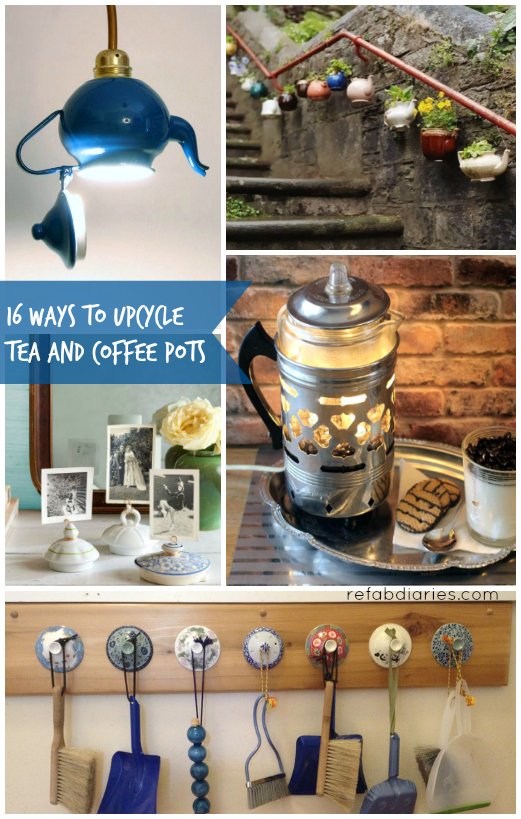The image is a vertical collage showcasing "16 Ways to Upcycle Tea and Coffee Pots," as indicated by a transparent blue banner with quirky white text. The top left photo features a blue teapot hanging upside down, repurposed into a light bulb fixture with its lid hinged open to let the light shine through—a quirky and creative design. Adjacent to it, in the top right, is a cement staircase adorned with red railings. Along these railings, around ten colorful teapots have been transformed into planters, each blooming with various flowers, adding a vibrant touch to the garden setting.

In the middle on the right, there's an old coffee pot turned into a light fixture, set on a tray in front of a brick wall. The tray also holds some cookies and a drink, possibly milk with chocolate. Below this, the bottom image spans the width of the collage and depicts a white wall with a wooden board used as a chair rail. Seven teapot lids of different shades of blue are affixed to the board, serving as hooks for small kitchen tools like whisk brooms and dustpans.

In the center left, a white table with a green base holds white flowers, positioned in front of a mirror with a dark wooden frame. In the foreground, three teapot lids have been cleverly adapted into photo holders, each displaying a black-and-white photograph. Another creative idea shown is a decorative cafetiere repurposed into a candle holder with tea lights inside, adding a cozy touch to the ensemble. The overall aesthetic combines blues, browns, and bright colors to showcase innovative and charming upcycling ideas.